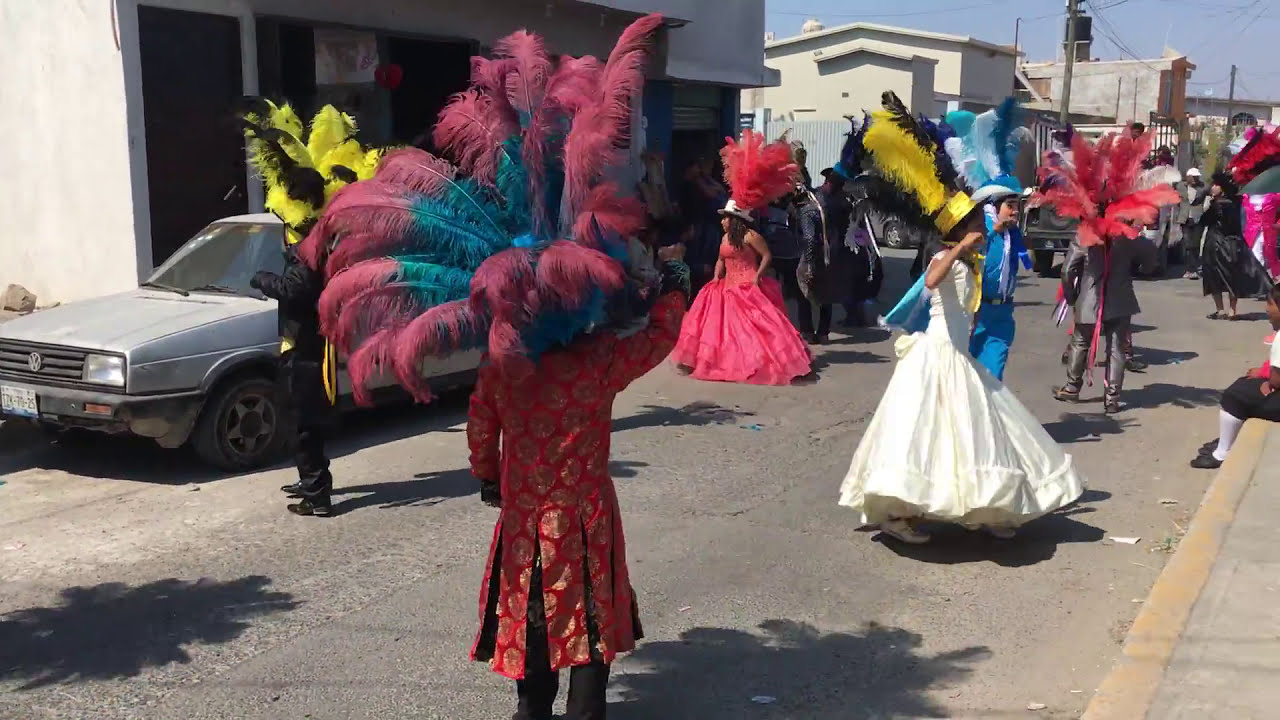The horizontal rectangular image captures a vibrant street parade set in an older part of a city. The street, showing signs of age with visible cracks and faint yellow curb paint, runs through the center of the picture. On the right side, part of a sidewalk is visible where someone is seated, watching the festivity. An old Volkswagen sedan, likely grayish-blue and bearing the classic VW logo, is parked on the left side next to a white stone building with numerous windows.

The parade is teeming with performers adorned in elaborate costumes and matching headdresses adorned with large, colorful feathers. Prominently featured in the middle foreground is a person facing away from the camera, dressed in a red and gold patterned coat with black pants, their hat brimming with pink and blue feathers. To their right stands a woman in a ruffled white dress paired with a black and yellow feathered headpiece. Beside her, a man in a turquoise suit accented with a blue and white feathered hat adds to the colorful display.

Further back, another woman in a dark pink dress with matching feathers and a man in a yellow and black feathered headdress enhance the scene's vividness. Beyond the immediate performers, the street hints at more participants in similarly elaborate attire. 

In the backdrop, older one-to-two-story buildings made of white and beige stone, along with utility poles, frame the clear blue sky above. The overall image conveys an old-world charm and a sense of festive celebration in a close-knit urban setting.